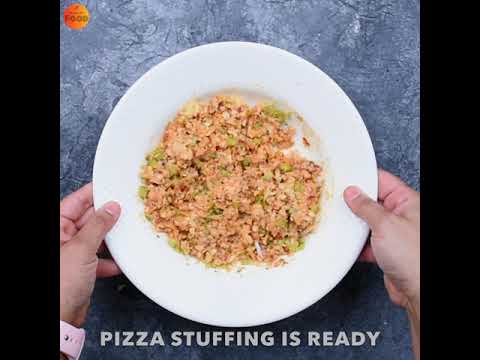In this image, we see a white glass plate being held by a pair of human hands, one on the right and one on the left, both visible from the forearms downward, with the left hand also showing a watch band. The plate, centered in the image, contains a mixture that appears to be pizza stuffing, featuring a brown and green color that gives it a somewhat mashed texture. The background is a slate gray or blue with a marbly texture, adding to the still, professional photography vibe, potentially from a cooking show or a YouTube tutorial. In the top left, there is a small red-orange circle with the word "food" inside, possibly indicating a food channel branding. Black borders frame the sides of the image, creating a square shape. At the bottom of the image, white text reads "pizza stuffing is ready," reinforcing the culinary theme of the scene.